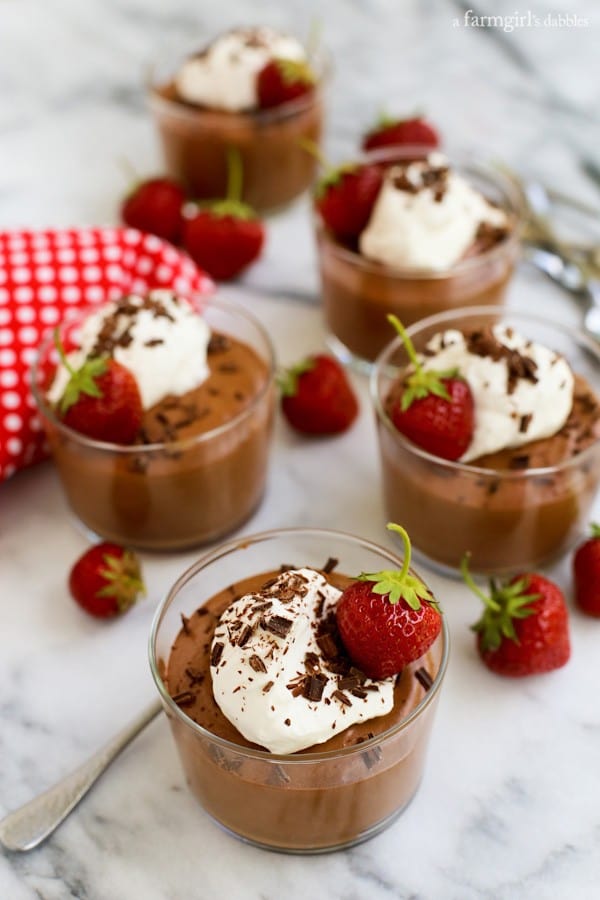Displayed on a white marble countertop, this image features five chocolate dessert cups with a focus on the cup nearest the viewer. Each transparent glass cup is filled with chocolate pudding, topped with white whipped cream and chocolate sprinkles, alongside a fresh, bright red strawberry. A red napkin with white polka dots and additional strawberries are scattered across the table. The text "a farm girl's dabbles," faintly visible as a watermark, is situated near the top right corner of the image. A partially obscured wooden utensil lies beside the closest dessert cup, adding an additional element to the detailed presentation.